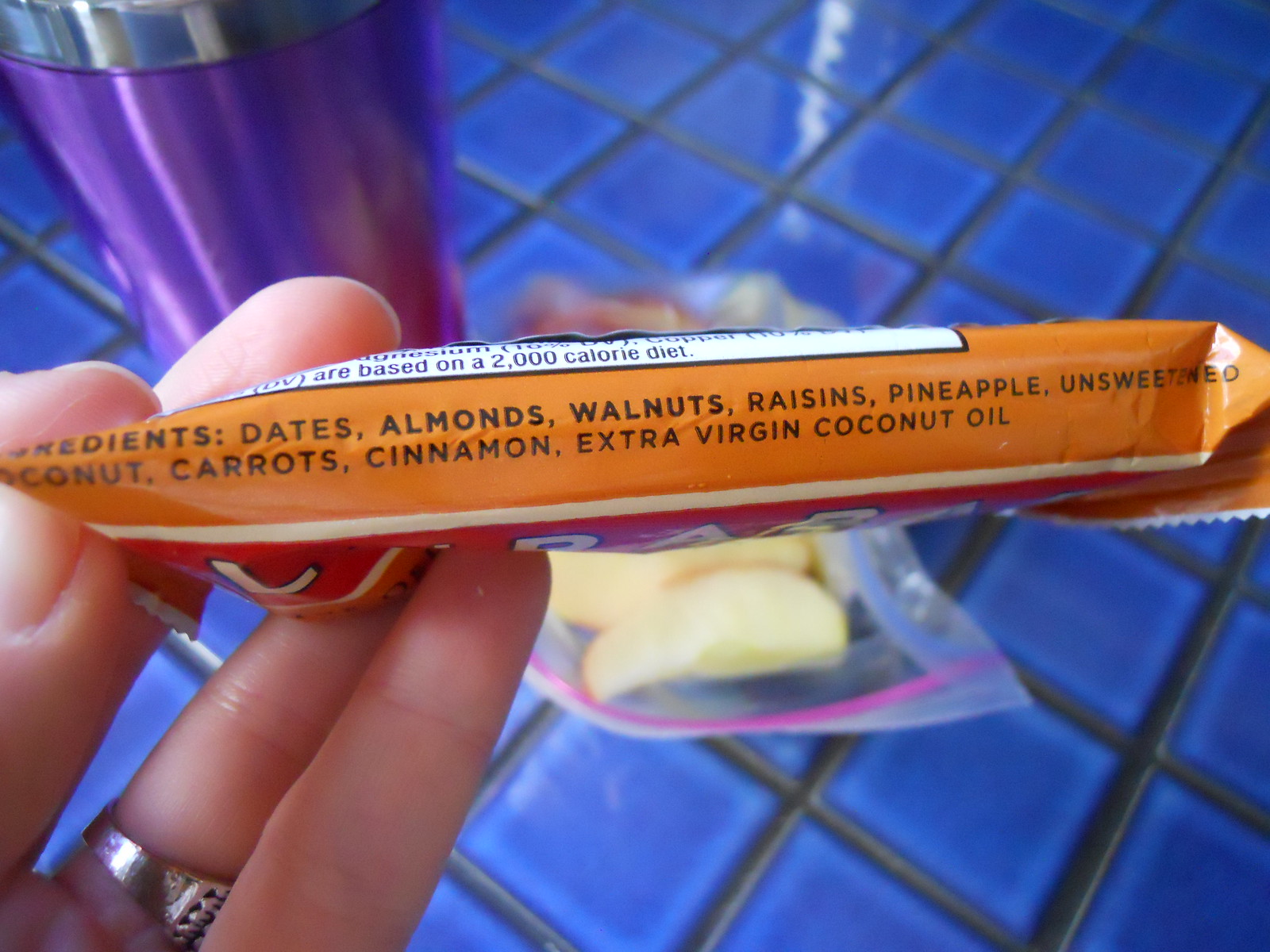In this vibrant color photograph, a hand emerges from the bottom left corner, holding up a granola bar in an orange package. The package, adorned with ingredients listed in black text, prominently reads "B-A-R." Situated above a blue tiled kitchen shelf, the scene is further enriched with a purple tumbler in the top left corner and an open Ziploc bag of light yellow fruit directly beneath the bar. The ingredients listed on the package include dates, almonds, walnuts, raisins, pineapple, unsweetened coconut, carrots, cinnamon, and extra virgin coconut oil. Bright overhead lighting casts highlights on the hand, the packaging, and the blue tiles, adding a touch of radiance to the composition.